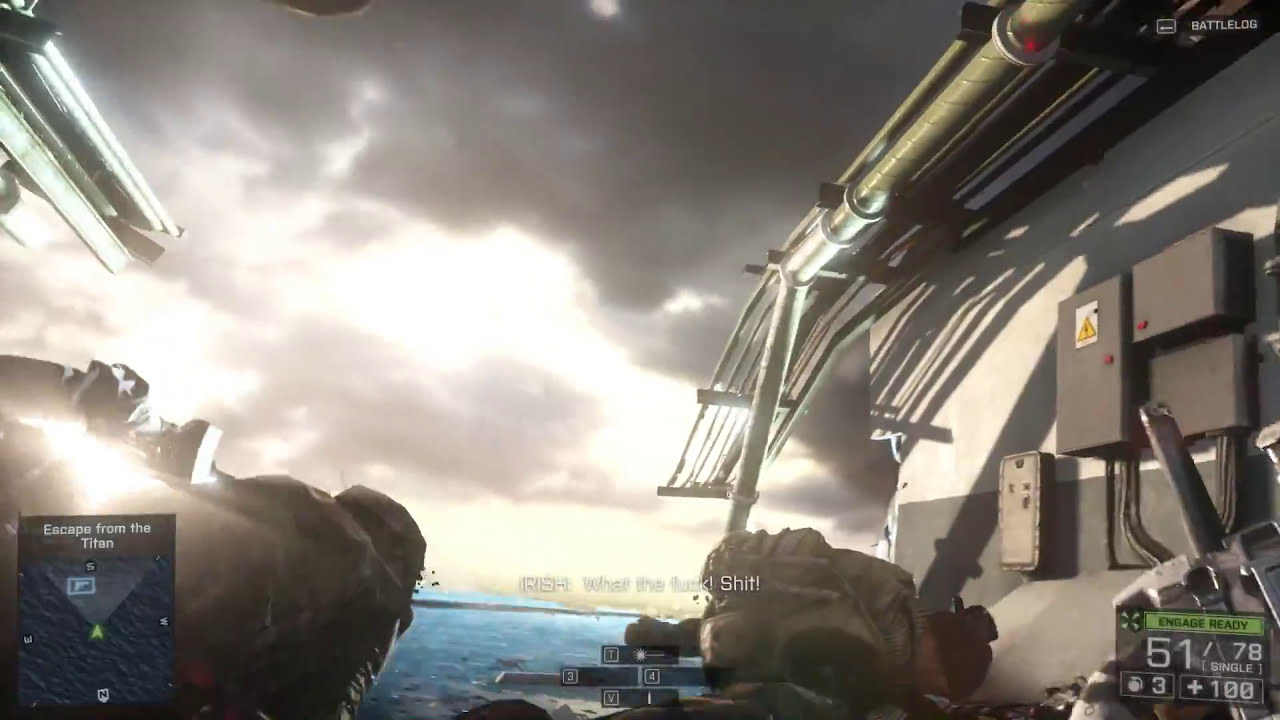The image is a screenshot from a video game, likely a shoot-em-up or first-person shooter game similar to Call of Duty. The setting is a military scene on a ship, with three soldiers visible. The background features an expansive, overcast sky with clouds emitting bright light, and a large body of rippled water. 

In the lower left corner, there is a map displaying the quest objective "Escape from the Titan," marked by a green arrow pointing south, surrounded by compass directions. The lower right corner shows the player's status: 51-78 bullets, 100 health points, and three grenades. Dialogue in the center of the screen includes exclamations like "Irish, what the fuck!" and "Shit, what a!"

The environment includes a metal or concrete wall on the left side, adorned with electrical boxes, lights, and a metal awning connected to pipes. A large gray wall with additional power boxes and a metal rail extending into a platform is visible on the right-hand side. There appear to be hands in leather gloves controlling equipment, suggesting a first-person perspective, possibly piloting a mech. The visual contrast between the bright sky and dark clouds adds to the dramatic atmosphere of the scene.